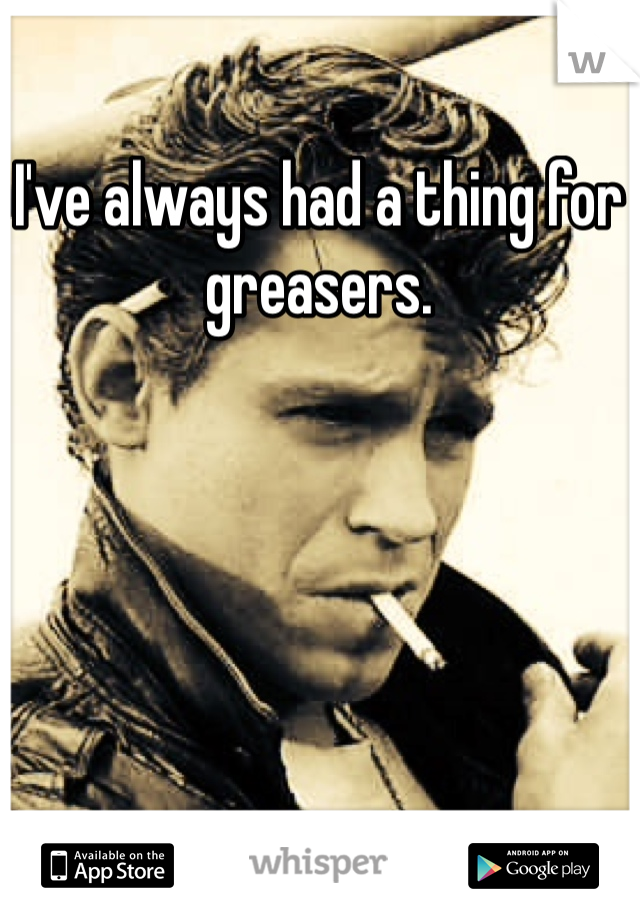The image appears to be an advertisement for the Whisper app, characterized by a distinctive retro aesthetic. At the very top, the image features white text with a black border that reads, "I've always had a thing for greasers." The photograph below exudes a classic greaser vibe reminiscent of the 1950s or 60s, showcasing a white male with voluminous, greasy, slicked-back hair. His expression is intense, with furrowed brows suggesting a sense of anger or focus. He sports a leather jacket with the collar up, and he seems to be tugging at it with one hand visible at the bottom right of the frame. The black-and-white image is tinged with an orange sheen, giving it an aged feel. The man has a cigarette in his mouth and another tucked behind his right ear. He is also wearing a white shirt beneath the leather jacket, and a hint of a silver necklace is visible. The background is an off-white, creamy color, brushed with the same orange hue. In the top right corner, there is a white square with a black "W." At the bottom, promotional logos indicate the availability of the Whisper app: on the left is a black and white icon for the App Store, alongside the text "Available on the App Store," in the center is the word "Whisper" in gray font, and on the right is the logo and text for "Android App on Google Play."